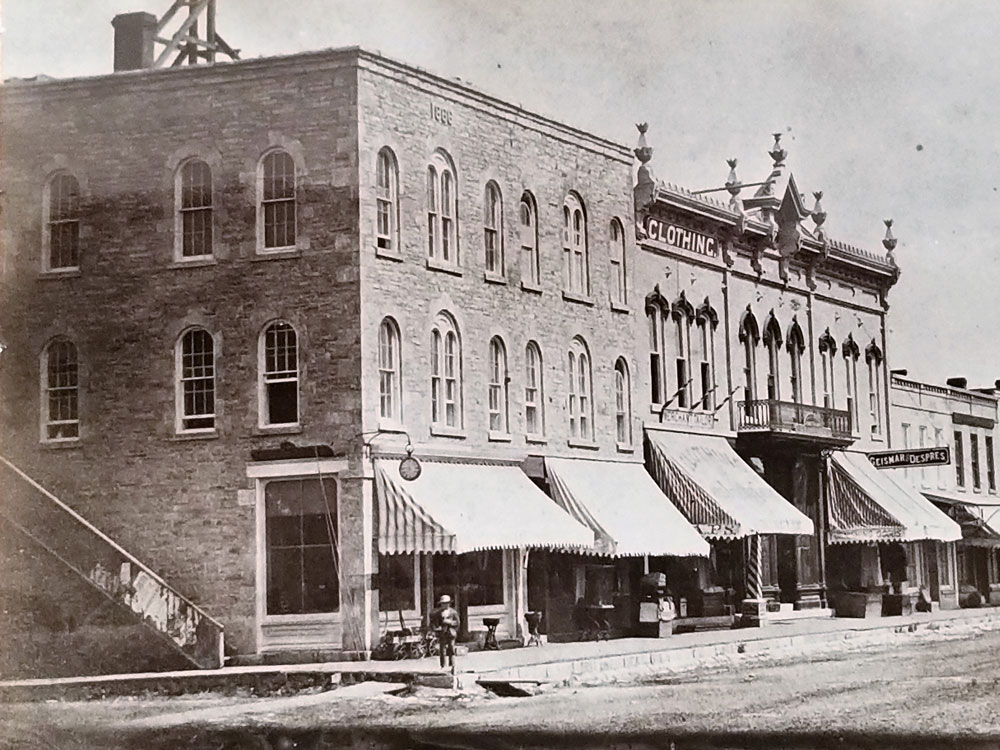This black and white photograph, likely taken around the late 1800s to early 1900s, captures a nostalgic scene of a small town. The focal point is a three-story brick building that stands prominently with a slight angle, revealing both its front and part of its side. The building, housing shops on the ground level, is characterized by large storefront windows and canvas awnings. The second and third floors feature rows of smaller windows. A wooden raised sidewalk fronts the building, and a person can be seen walking at the corner, adding to the timeless appeal.

Adjacent to the main building are two additional structures. The first neighboring building is a slightly shorter two-story structure, dawned with signage indicating "CLOTH INC" at the top and featuring more storefront windows and awnings. The final adjoining building is another two-story property with windows and an awning, though notably shorter in height compared to the others. Details like a clock on the corner, an external staircase on the side, and a somewhat cloudy sky in the background contribute to the vintage, grainy esthetic of this historic streetscape photograph.